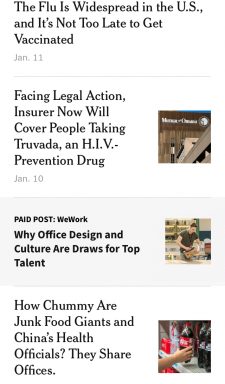The image displays several sections of information organized in a column format:

1. At the top, bold, black text reads, "The flu is widespread in the U.S." Below this, another line states, "It's not too late to get vaccinated." The date "JAN. 11" is printed in a light gray color.

2. The next section addresses legal matters with the heading, "Facing legal action, InsureNow will cover people taking Truvada, an HIV-prevention drug." This text is also black, and to the side is an unidentifiable icon. The date for this section is "JAN. 10."

3. The following boxed area, marked as a "Paid Post," features slightly lighter text, reading, "WeWork: Why office design and culture are draws for top talent." This section includes an image of a person engaged in a task.

4. The final section poses a question: "How chummy are junk food giants and China's health officials?" followed by the statement, "They share offices."

The overall visual structure uses varying shades of text to differentiate sections and dates while incorporating images and icons to enhance the contextual information.